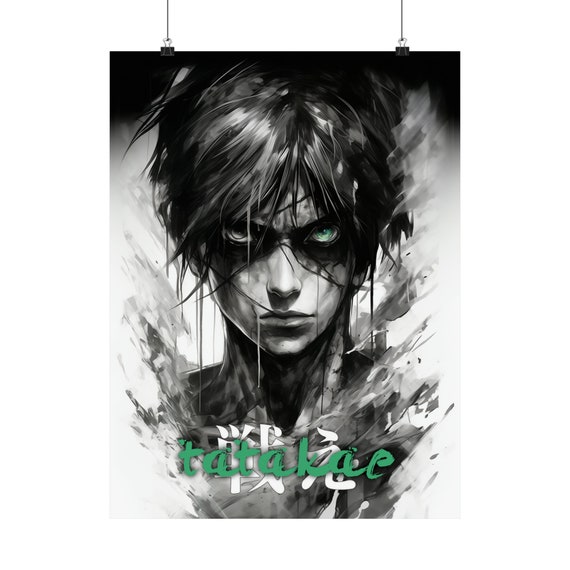The black-and-white digital artwork portrays a broody, enigmatic character with dark, shadowy eyes, staring directly forward. The figure has short, ruffled ear-length black hair with messy bangs partially obscuring their eyes, which are highlighted by pronounced dark shadows or eye shadow. The bust of the character is surrounded by abstract smoke shapes, created using expressive, messy brush strokes. Green text above the figure reads "Tata Kai," accompanied by Asian characters underneath. The overall style resembles Japanese anime, with an unfinished, sketch-like quality characterized by numerous black lines extending from the bust. Despite the character's neutral facial expression and minimalist black mask, there's a palpable, dark aura to the image.